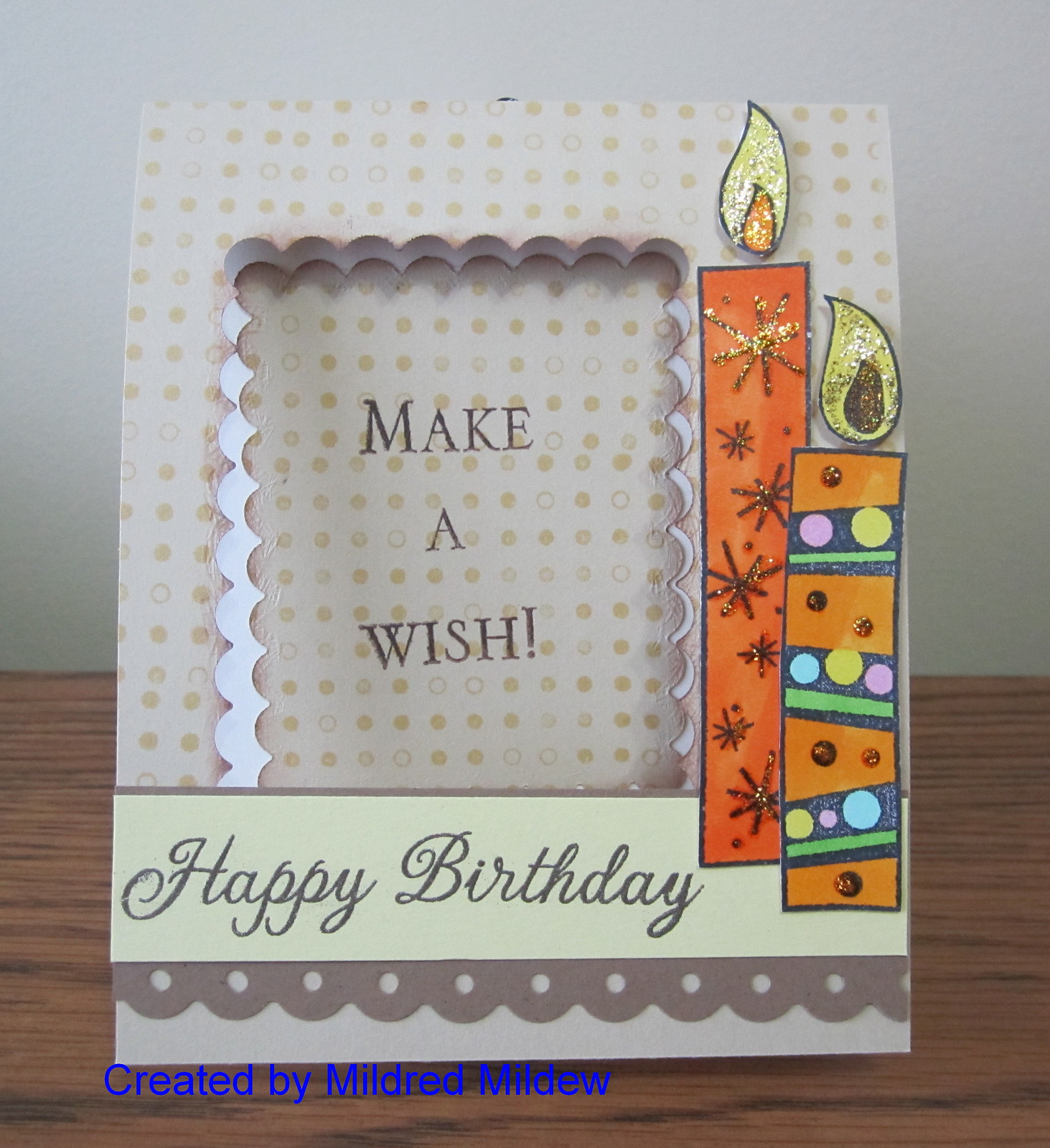The photograph showcases a detailed greeting card positioned on a brown table against a white wall. The card features a predominantly white background adorned with numerous gold polka dots. Its unique design incorporates a double scallop cutout on the front, through which the phrase "Make a Wish" is visible in capital letters with an exclamation point, giving a window-like effect. To the right of this central message are two decorative birthday candles. The left candle is orange with gold glitter and snowflake-like shapes, while the right one displays a multi-colored pattern with blue and yellow stripes interspersed with dots, and yellow flames are depicted atop both candles. Below "Make a Wish," a gray script spells out "Happy Birthday" on a white rectangular band. At the very bottom right corner of the card, blue text reads "Created by Mildred Mildew." This intricate design captures an artistic birthday greeting in a stationary format.